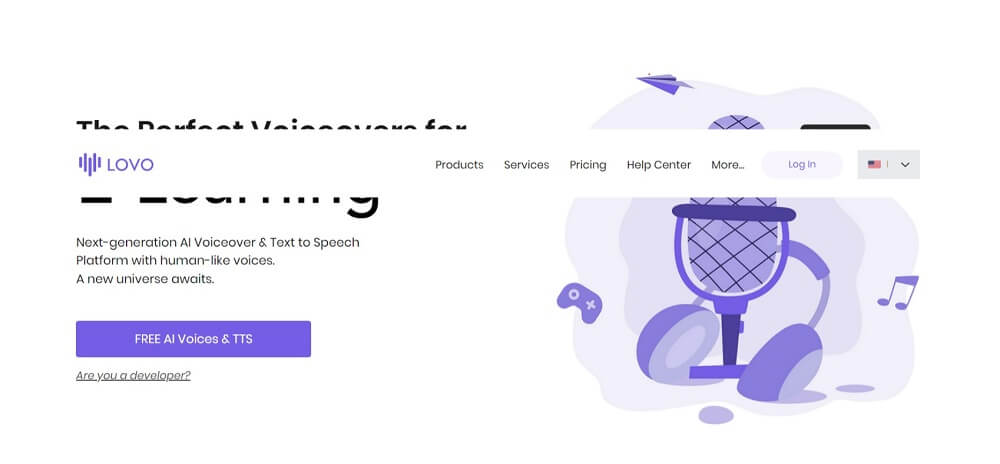The image is a screenshot of a white-background website's upper section. At the top, a partially visible header reads, "The Perfect," but the text is obscured by a banner overlay. Prominently featured is a stylized purple heart formed by lines of varying lengths with the text "LOVO" in bold, purple, capital letters.

Below the header, a horizontal navigation menu displays options: "Products," "Services," "Pricing," "Help Center," and "More," the latter represented with an ellipsis (…). A "Login" button is to the far right, colored in light purple with purple text. Adjacent to it, a gray square with an American flag and a dropdown menu is present.

On the left side, black text reads, "Next-generation AI voice-over and text-to-speech platform with human-like voices." The text features hyphens in "next-generation" and "human-like." Directly beneath this, a purple clickable link states, "Free AI Voices and TTS," followed by an underlined question, "Are you a developer?"

On the right side, under the navigation menu, the image displays a purple microphone surrounded by headphones, a gaming remote control, and a music note icon, emphasizing the platform’s functionality and versatility.